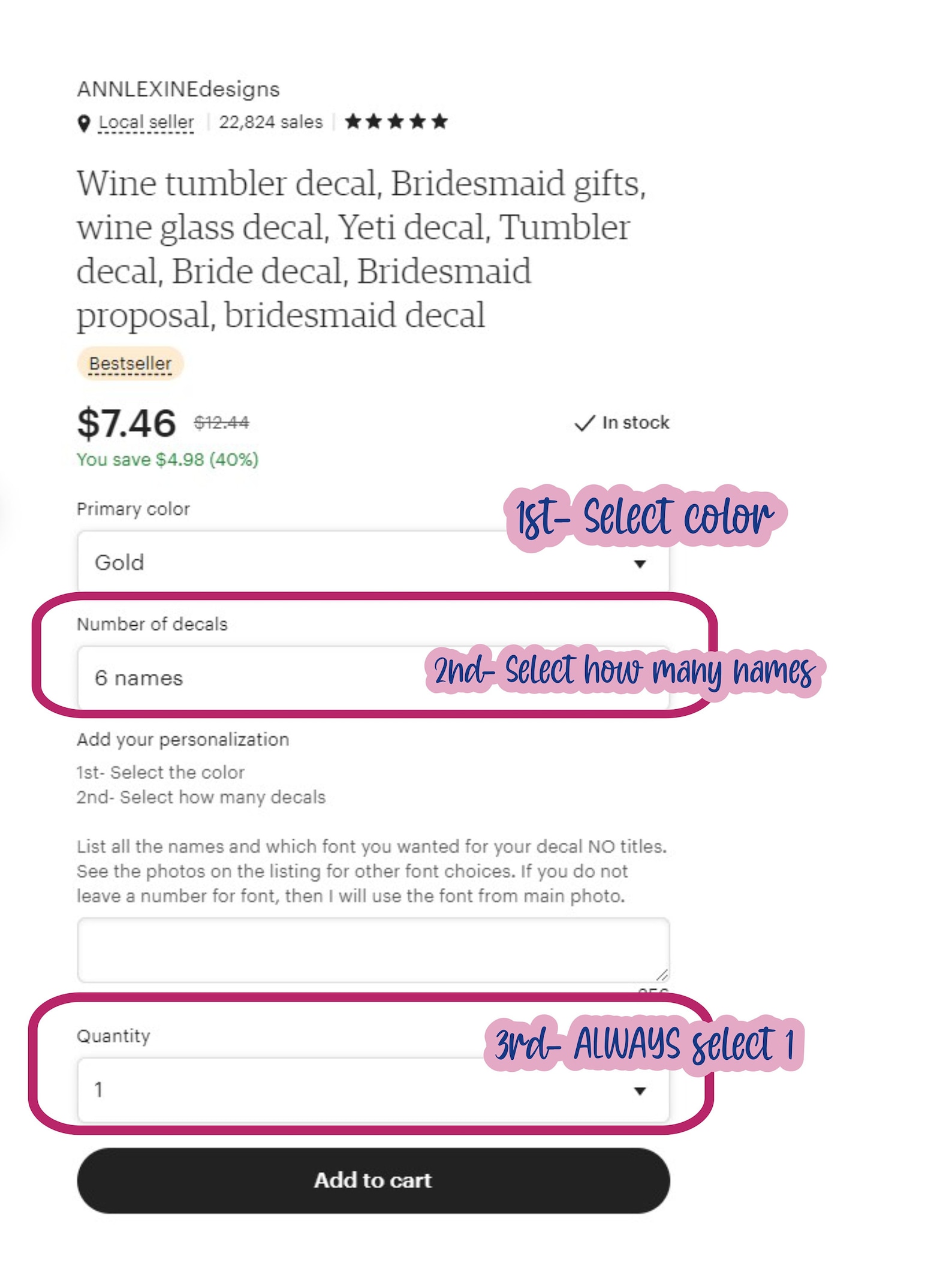On a product page from Anne Lexine Designs, the featured item is a customizable Wine Tumbler Decal, ideal for Bridesmaids Gifts, Wine Glass Decals, Yeti Decals, Tumbler Decals, Bride Decals, Bridal Proposals, and Bridesmaid Decals. The current price of the decal is $7.46, marked down from the original price of $12.44, offering a savings of $4.98 or 40%. Shoppers can select a color for their decal, with gold being one of the available options. They can also specify the number of decals needed and provide the names to be included. Below this, there is a field to adjust the quantity. Instructions overlayed on the right-hand side within a pink bubble with blue font guide users through the purchasing process: first, select the color from the dropdown menu; second, select the number of names; third, always select the quantity as one; and finally, add the item to their cart.